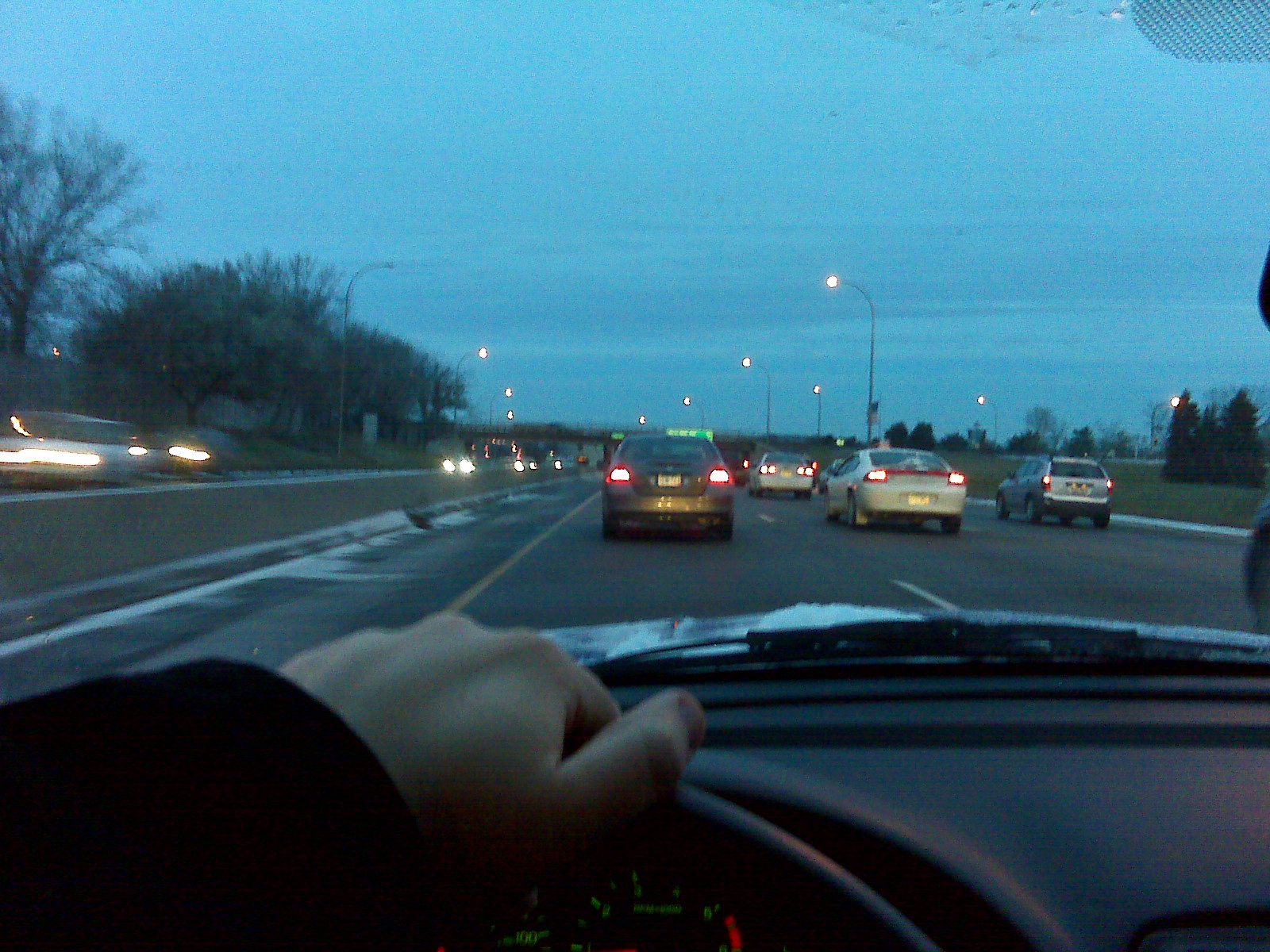The image captures a scenic yet bustling highway scene from the perspective of someone driving an older, smaller car. The driver’s left hand, dressed in a long-sleeved black shirt or jacket, is seen gripping the top of the steering wheel. The car's dash and partial odometer are visible just behind their hand. It appears to be early evening, as the sky is a deep blue and the streetlights are illuminated, casting a subtle glow over the surroundings. The highway, a three-to-four lane thoroughfare separated by a grass median and a cement curb, is busy with vehicles. In the driver's lane, brake lights indicate slowing traffic, likely rush hour congestion. Ahead, multiple cars span the visible lanes and more headlights can be seen in the opposite direction, highlighting the dense traffic flow. The view also includes a few trees, grass, and some houses on the side of the highway, along with a distant bridge that adds depth to the image. The windshield wiper peeks into the frame, reminding viewers of the everyday nature of this moment on the road.